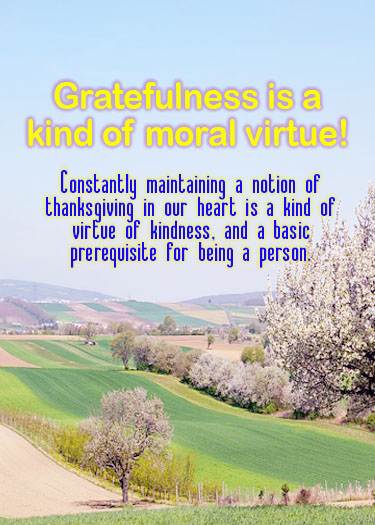A detailed map poster features an inspiring message about the importance of gratitude, prominently displayed in vibrant colors. At the top, in bright yellow text with an exclamation point, it declares: "Gratefulness is a kind of moral virtue!" Below, in bold blue text, it elaborates: "Constantly maintaining a notion of Thanksgiving in our heart is a virtue of kindness and a basic prerequisite for being a person." The background of the poster is adorned with picturesque green rolling hills, dotted with trees, and framed by majestic mountains. Above it all, a clear blue sky stretches seamlessly, adding to the serene and uplifting atmosphere of the poster.